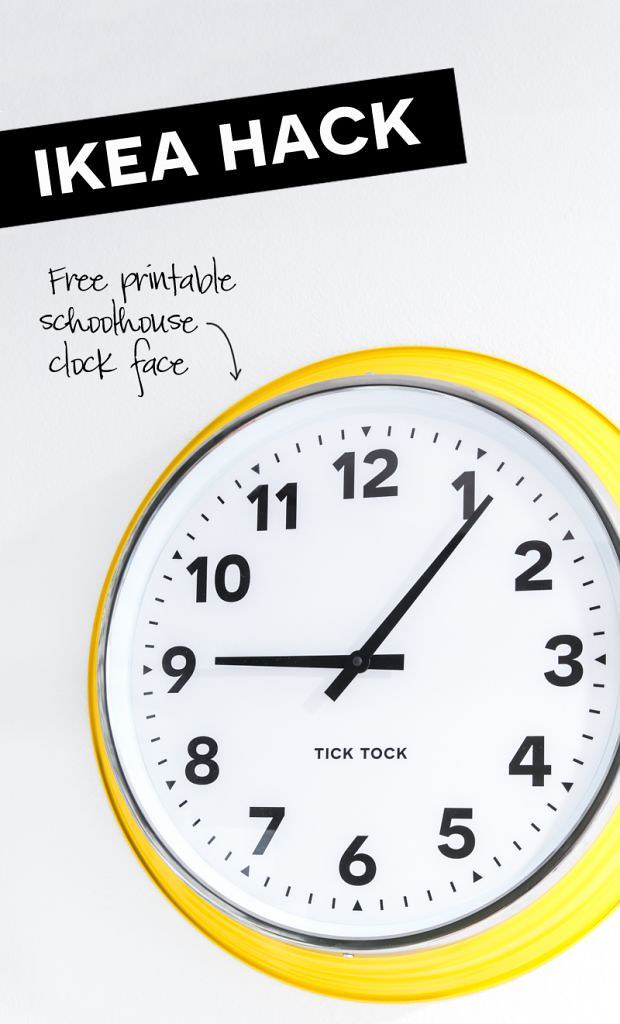This promotional image is likely part of a brochure or website advertisement featuring an IKEA hack. The black banner at the top of the image announces "IKEA Hack." Directly below this banner is the text "Free Printable Schoolhouse Clock Face." An arrow points downward to a clock, which appears to be intended for wall mounting. The clock has a white face adorned with black numbers and black hands, with the words "TIK TOK" printed in its lower middle section. Surrounding the clock face is a yellow bezel. The image encourages viewers to download and print this decorative schoolhouse clock face, which, despite not being functional as a timepiece, serves as a visually appealing DIY project.